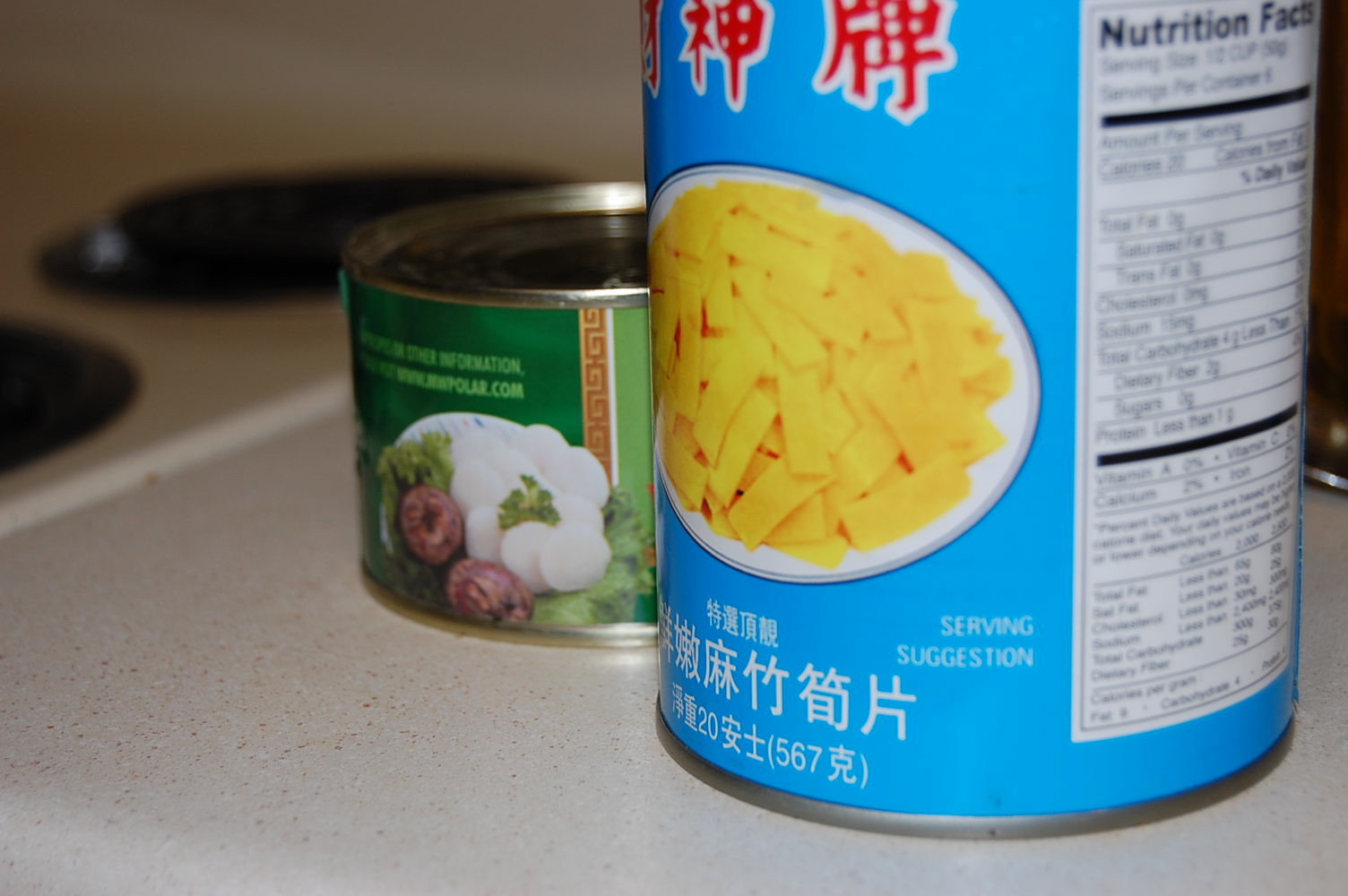In this rectangular image oriented horizontally, the focal point is on two cans of food placed on a countertop. The foremost can, positioned on the right side of the image, is upright and predominantly blue. This blue can features a visual of small rectangular yellow noodles on a plate, indicative of its contents. The label displays characters that appear to be either Chinese or Japanese, alongside an English phrase "serving suggestion." Towards the bottom, the numbers "20" and "5, 6, 7" are visible. A white label with black text indicating nutritional facts is present but largely illegible except for the title. The base of this can is accentuated with a metallic trim.

Behind the blue can and slightly obscured by it, there is a second can, roughly half the height of the first one. This smaller can is primarily green, hinting at a different type of food product inside.